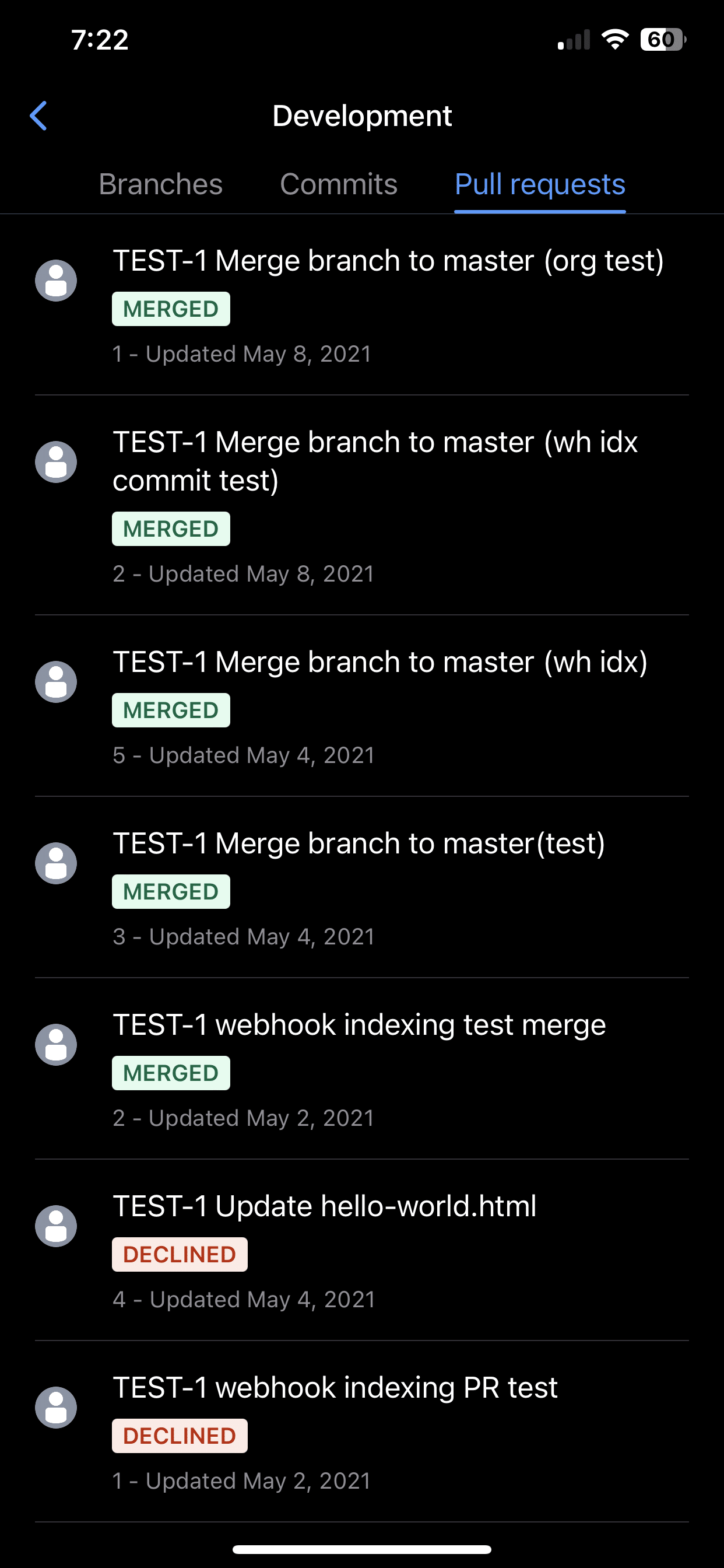The image portrays a mobile phone screen displaying a development interface on a black background. The top section prominently shows the title "Development" with three navigational tabs underneath labeled "Branches," "Commits," and "Pull Requests." The "Pull Requests" tab is highlighted in blue, while the other tabs are in standard gray, indicating the current focus is on pull requests.

Below the tabs, a series of entries detail various pull request activities:

1. **Entry 1:**
   - **Description:** "Test one - merge branch to master"
   - **Author:** org test
   - **Status:** Merged
   - **Date:** May 8th, 2021
   - **Icon:** Small person icon

2. **Entry 2:**
   - **Description:** "Test one - merge branch to master"
   - **Author:** WHIDX
   - **Commit Message:** "Commit test"
   - **Status:** Merged (Green text)
   - **ID:** #2
   - **Date:** May 8th, 2021

3. **Entry 3:**
   - **Description:** "Test one - merge branch to master"
   - **Author:** WHIDX
   - **Commit Message:** "merged"
   - **ID:** #5
   - **Date:** May 4th, 2021

4. **Entry 4:**
   - **Description:** "Test one - merge branch to master (test)"
   - **Author:** Unknown
   - **Status:** Merged
   - **ID:** #3
   - **Date:** May 4th, 2021

5. **Entry 5:**
   - **Description:** "Test one - webhook indexing test"
   - **Status:** Merged
   - **ID:** #2
   - **Date:** May 2nd, 2021

6. **Entry 6:**
   - **Description:** "Test one - update hello world.html"
   - **Status:** Declined (Red text)
   - **ID:** #4
   - **Date:** May 4th, 2021

7. **Entry 7:**
   - **Description:** "Test one - webhook indexing PR test"
   - **Status:** Declined (Red text)
   - **ID:** #1
   - **Date:** May 2nd, 2021

Additional information at the bottom right corner of the screen indicates the time as 7:22, and the battery level is approximately 60%.